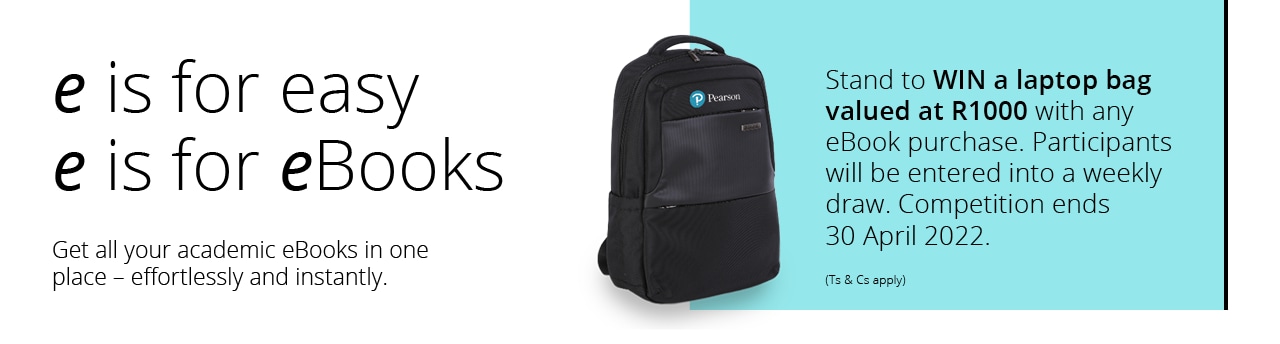The advertisement features a promotion for a black backpack displayed prominently in the center against a split white and blue background. The left side of the ad, set against a white backdrop, contains bold black text that reads: "E is for Easy, E is for eBooks." Beneath this, in smaller text, it states: "Get all your academic eBooks in one place, effortlessly and instantly." 

Adjacent to this, the right side of the ad has a turquoise background with centered black text that announces: "Stand to win a laptop bag valued at R1000. With any eBook purchase, participants will be entered into a weekly draw. Competition ends 30 April 2022." At the bottom, there is small print noting, "T's and C's apply."

The black backpack, situated in the middle, features the brand name "Pearson" along with a small turquoise emblem, bridging the ad’s two halves. The backpack appears to have multiple compartments, a top handle, and likely shoulder straps, although they aren't clearly visible.